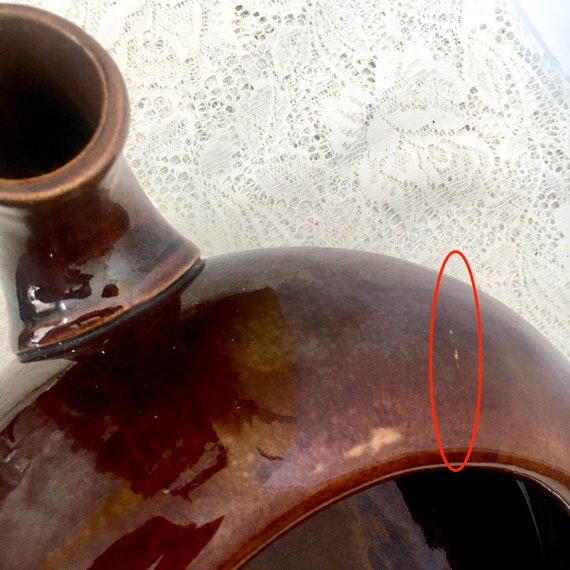The photograph provides a detailed, overhead view of a dark brown, shiny, ceramic teapot, positioned on an intricate, white lace doily. The teapot, which has a distinctive reflective glaze, appears to show the reflections of the photographer, creating a dynamic and textured surface. The doily beneath it is reminiscent of vintage, finely crocheted tablecloths, enhancing the elegance of the scene. A notable feature of the teapot is a red oval-shaped circle highlighting a minor defect—a small scratch or nick—located adjacent to the spout, just below the area where the cover would sit. This red circled area draws attention to the blemish, possibly indicating the photograph's use for a detailed listing or customer inspection scenario. The image shows the teapot's opening, partially exposing its dark, reflective interior. Overall, the composition focuses on showcasing the teapot's condition and the subtle imperfections on its surface.